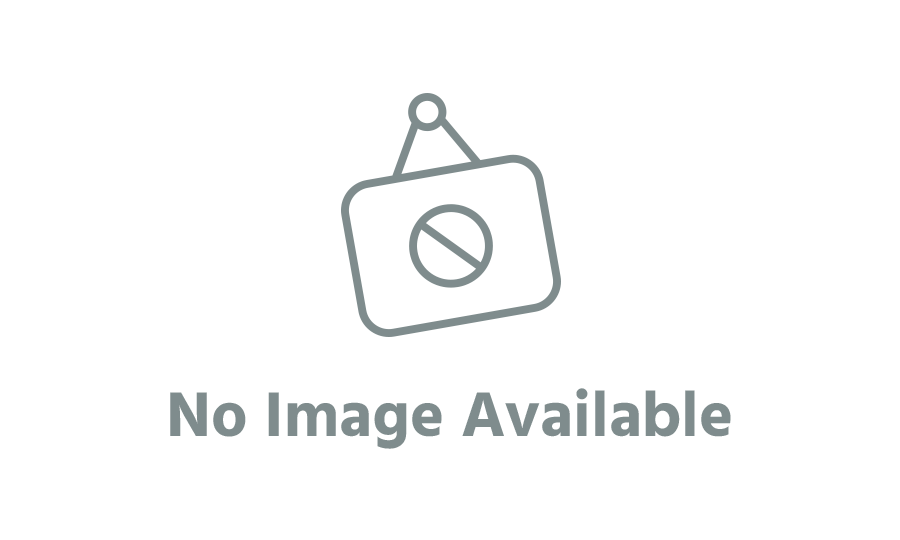The image is an AI-generated fantasy illustration of a young blonde woman with classic, overly idealized features such as a heart-shaped face, large bright blue eyes, a perfect nose, and petite lips. She exudes an angelic aura with her porcelain-like fair skin and is gazing to the right. Her long, thin blonde hair cascades around her, interwoven with strands of blue, pink, cyan, magenta, gold, blue, purple, and yellow. She is adorned with a headdress featuring a round gold medallion with a see-through gem at the front, surrounded by flowers and feathers that extend across the top of the image. Her attire is a luxurious turquoise and gold top with gold filigree designs around the sleeves and collar, which is decorated with little arches and intricate filigree patterns. The background is vibrant and swirling, filled with February-themed ornamentation in shades of gold and blue, wrapping around her and integrating seamlessly with the elements in the foreground, including her flowing hair and the decorative flowers.